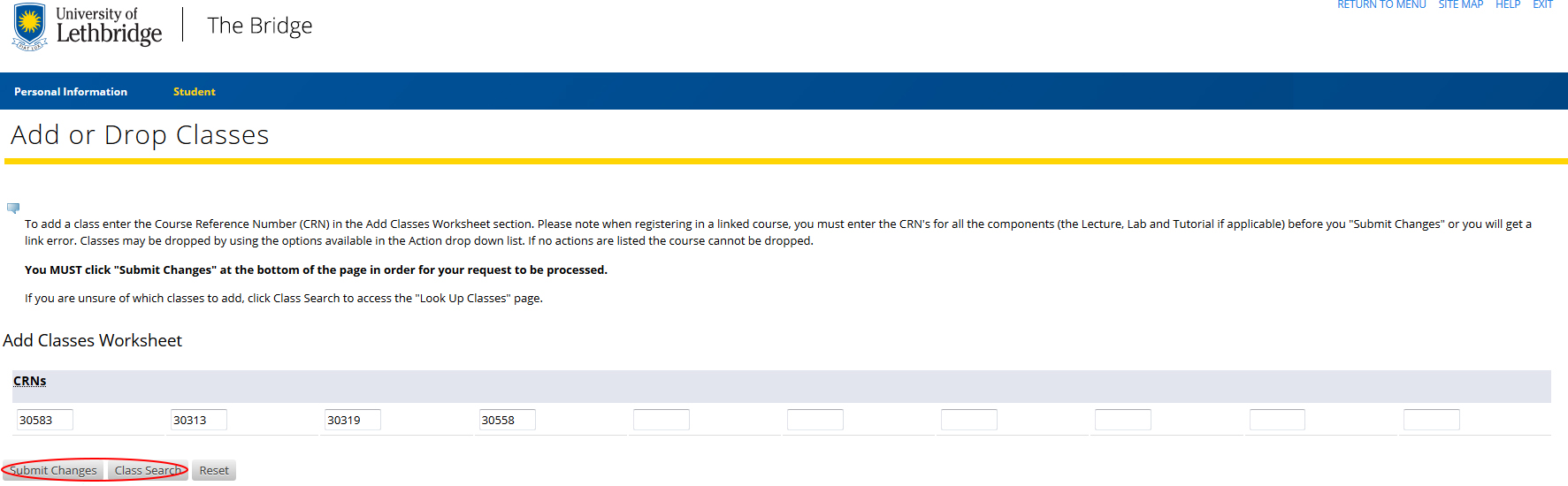This is a detailed screenshot of a horizontally-oriented interface, either from a PC or a tablet, showcasing a partial view of a website for the University of Lethbridge. The background is predominantly white with navy blue text and elements. At the top of the page, a heavy navy blue line serves as a border, just below which the text "University of Lethbridge" is prominently displayed. To the left of the text is a shield emblem featuring blue, yellow, and gold on a white background.

Above the shield, the University’s name is printed in navy blue, while to the right, in a faded font, the word "bridge" can be seen. The heading at the top of the page reads "Add or Drop Classes," indicating that this section is dedicated to managing course enrollments. 

Additionally, there is a red-circled item towards the top, suggesting that the screenshot might be part of a tutorial or a guided walk-through for new users, or it could be highlighting a specific action point. The page contains multiple lines of faint blue text, and below the "Add Classes Worksheet" header, a pale blue line is visible, further dividing the content.

The intricate design and detailed instructions indicate this is a functional part of the university's online system for course management.